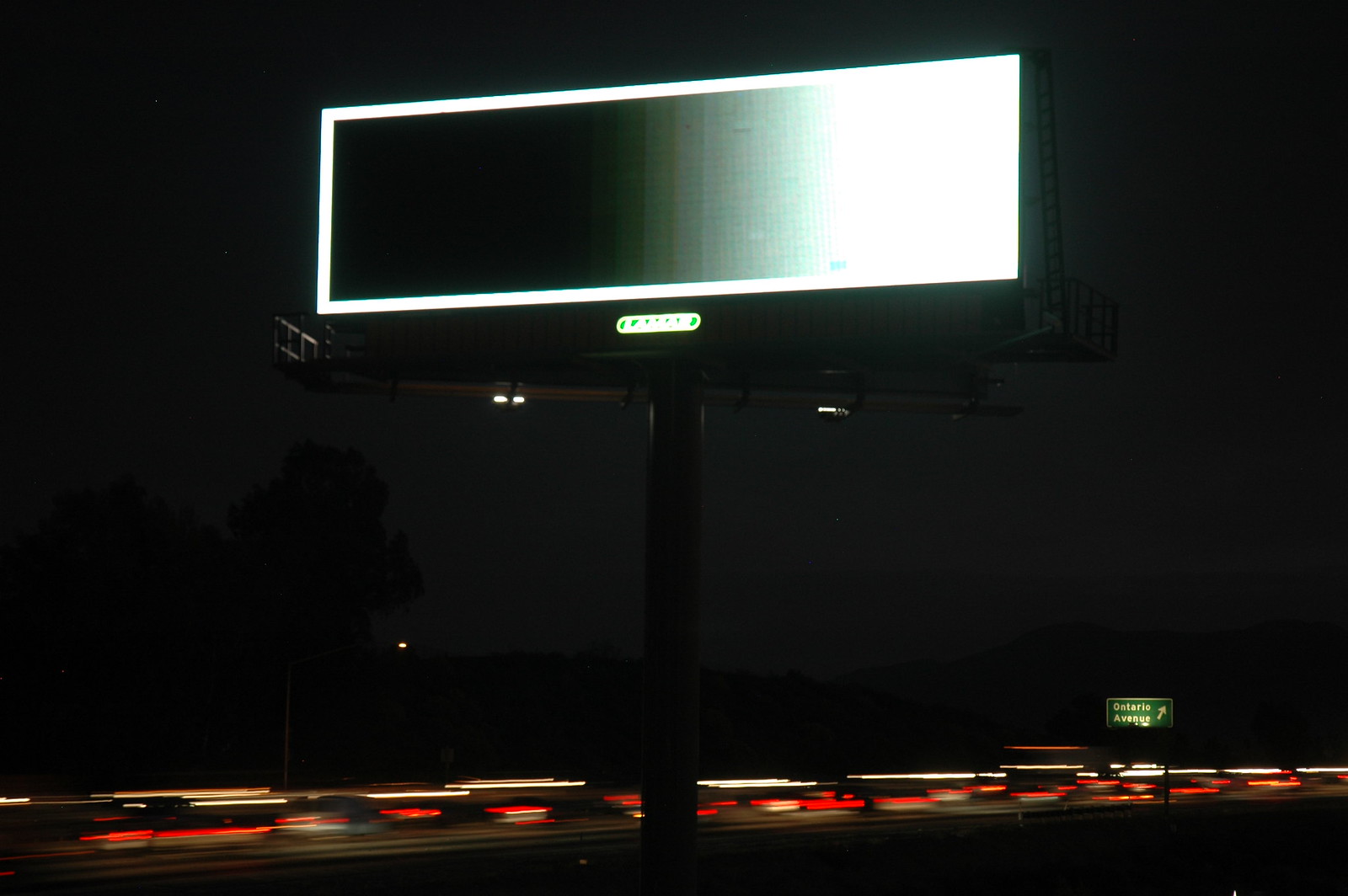The image captures a sleek, new digital billboard prominently displayed above a bustling highway at night. The billboard, resembling a massive flat-screen TV with a distinctive white edge, is mounted on a thick, black pole. The support structure includes a black box platform and scaffolding on either side, partially obscured by the night. Faint lights beneath the billboard illuminate an oblong sign, the text of which is unreadable. Below, the highway is alive with the glow of car headlights and taillights. A green exit sign is visible in the background, and a sparse outline of trees borders the road, completing the nocturnal scene.